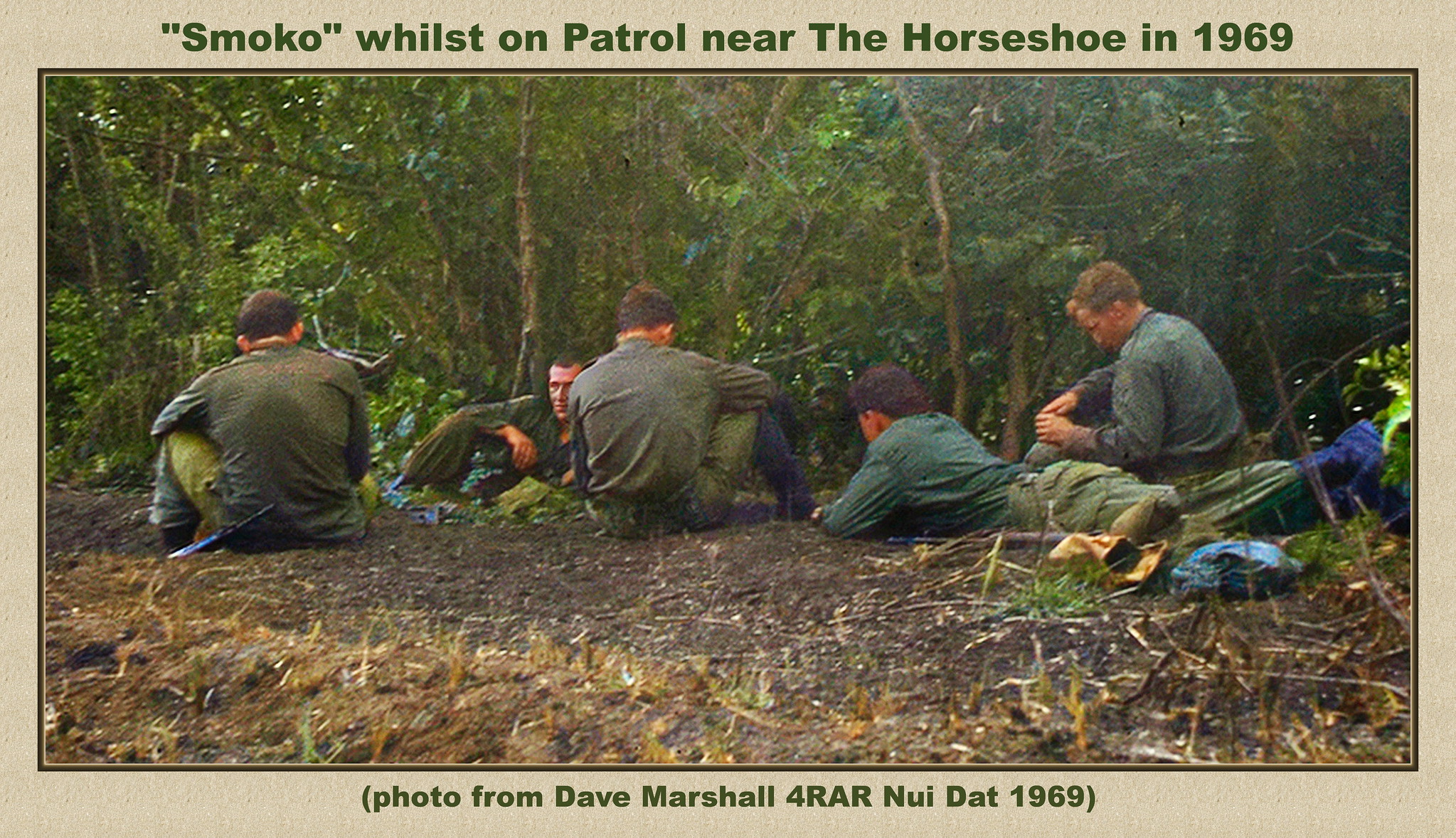The postcard features a photograph bordered by beige with green lettering at the top that reads, "Smoko whilst on patrol near the Horseshoe in 1969." The image is credited at the bottom, "photo by Dave Marshall for RAR Nui Dat 1969." The scene captures five soldiers, mostly with their backs turned, clad in dark green military attire, seated or lying on the cleared, earthy ground. The second soldier from the left is the only one partially facing the camera. They are gathered with scattered camping supplies to the right and what appears to be a blue can between the first and second soldier on the left. The background is a dense forest with an array of trees and shrubbery. This image, likely from the Vietnam War era, depicts a moment of rest amidst a patrol.